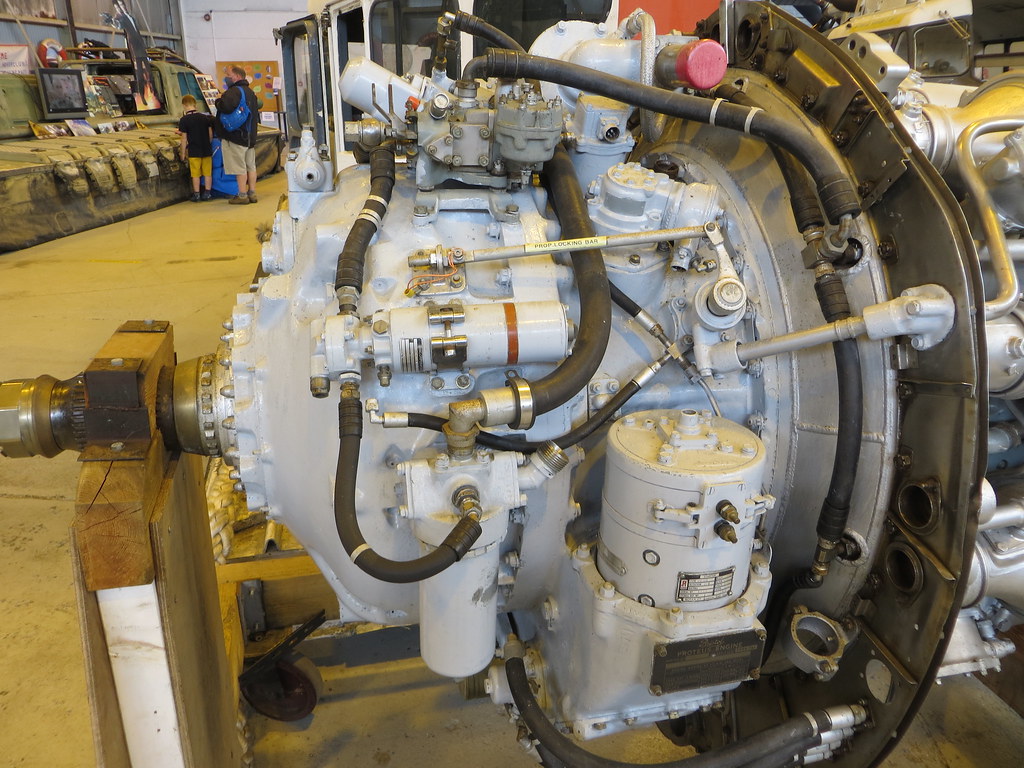This image showcases a large, industrial device positioned centrally amidst a complex network of pipes and tubes of varied colors, including black, white, and silver. The device features a long cylindrical structure adorned with multiple bucket-like attachments, valves, and tubes. At its base and to its right are white can-like tubs. The setting suggests a factory or an indoor industrial environment with a cement floor. In the background, two figures—a man and a child, presumably father and son—stand on the upper left, with the child on the left and the man, carrying a blue bag, on the right. They appear to be observing screens displaying additional equipment and machinery, contributing a sense of human scale and anomaly to the otherwise heavily industrial scene.